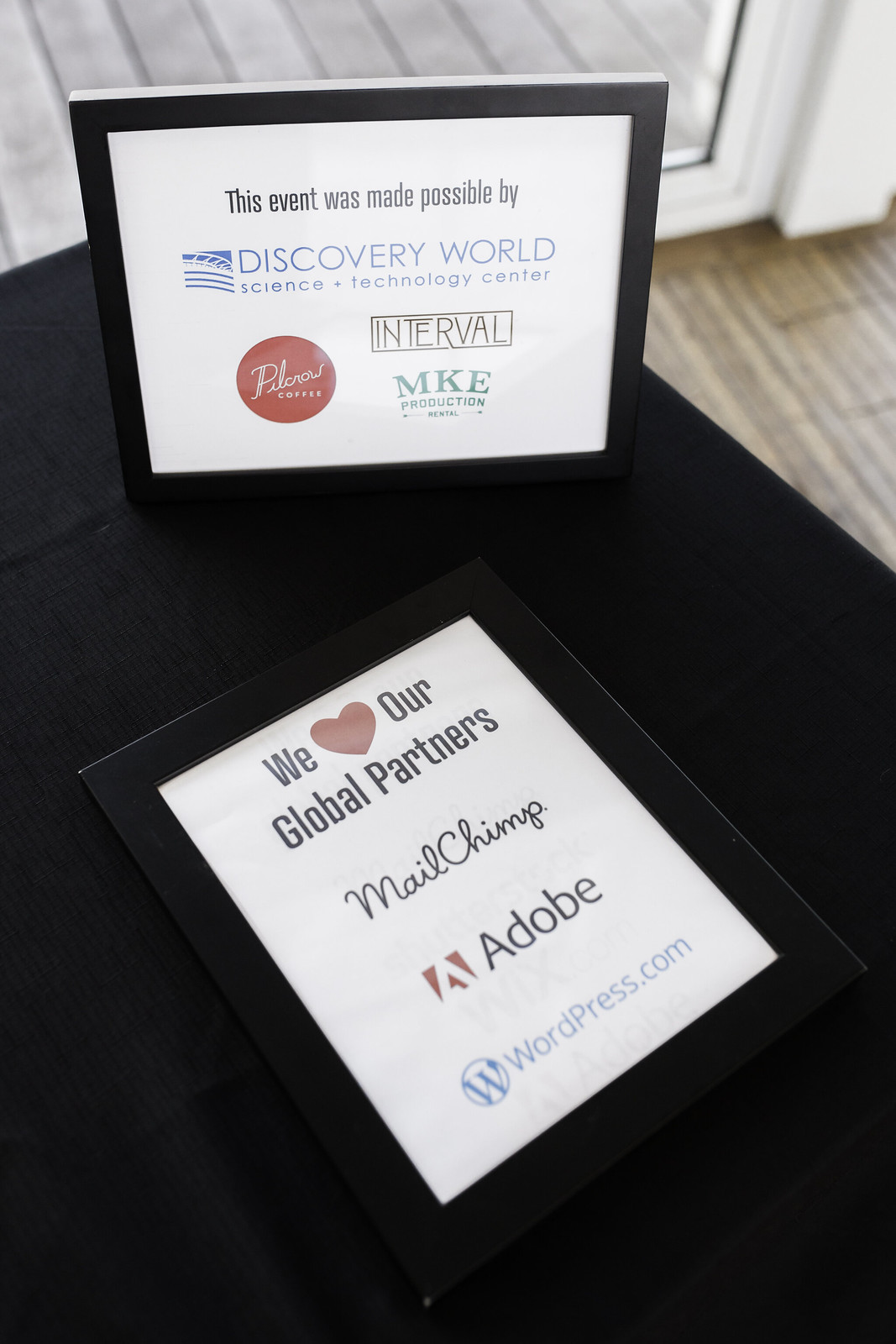In this photograph taken from above, we see a black tabletop covered with a black tablecloth, situated against the backdrop of a wooden floor and a sliding glass door. Two framed certificates are placed on the table. The bottom frame, laying flat, contains a white paper that reads "We", followed by a large red heart, and then "Our Global Partners." Below that, the names "MailChimp" in cursive, "Adobe" with a red Adobe symbol, and "WordPress.com" in blue lettering are displayed.

The second frame, which is standing, is positioned above the first in the photo. It also has a white piece of paper, beginning with the text "This event was made possible by" in black font. Below this, in blue lettering, it says "Discovery World Science Technology Center." There is a red circular logo towards the bottom left, though the text within it is unreadable. To the right of the red circle, the word "Interval" appears inside a black-bordered rectangle, and below that, in green font, it says "MKE Production."